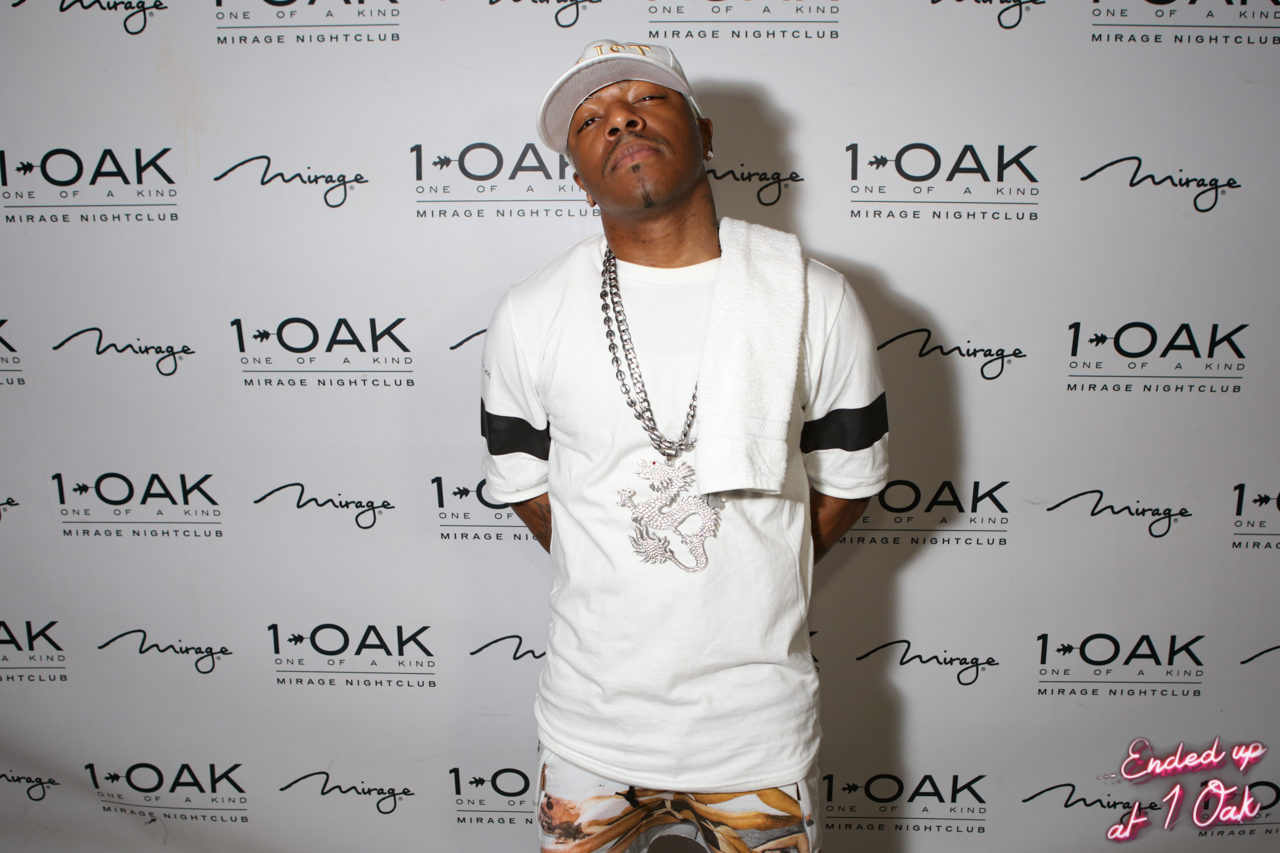In front of a patterned white banner featuring alternating "One Oak" in bold black capital letters and "Mirage" in cursive, an African-American man poses for the camera. The banner, indicative of a high-profile event, also includes the phrase "one-of-a-kind Mirage nightclub" repeatedly from top to bottom. In the lower right corner, in pink cursive font, it reads "ended up at one oak."

The man, who resembles the rapper Sisqo, stands with a confident yet coy expression, subtly scowling. He wears a white baseball cap, a white short-sleeve t-shirt with black stripes around the sleeves, and a striking necklace featuring a large silver dragon pendant hanging down to his stomach. His dark skin contrasts with his outfit, which includes white stretch pants adorned with a brown pattern. He also sports a thin mustache, slight chin hair, and holds his hands behind his back, casting a noticeable shadow due to the bright lighting.